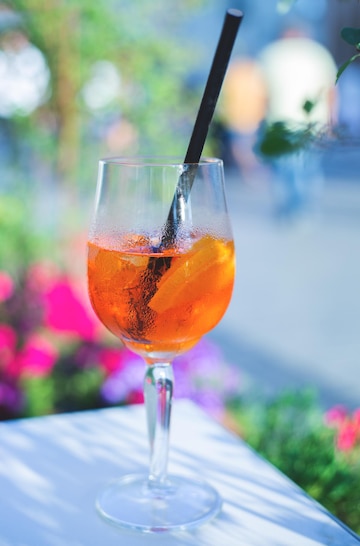This vibrant image captures a close-up of a wine glass filled with a refreshing orange beverage, possibly iced tea or a citrus drink, adorned with a slice of orange and a black straw. Resting on a white tablecloth outdoors under the bright sun, the melting ice within the drink suggests a warm, sunny day. In the blurred background, lush green foliage and clusters of pink flowers add to the picturesque setting. There are also subtle human elements: a man in a white shirt with blue jeans is seen walking away, accompanied by another in a yellow shirt and jean shorts. To the right, just the edge of another blue shirt is visible, and the top left corner features cascading vines with interspersed flower baskets. This detailed scene exudes a serene and refreshing atmosphere, perfect for a simple, relaxing day.